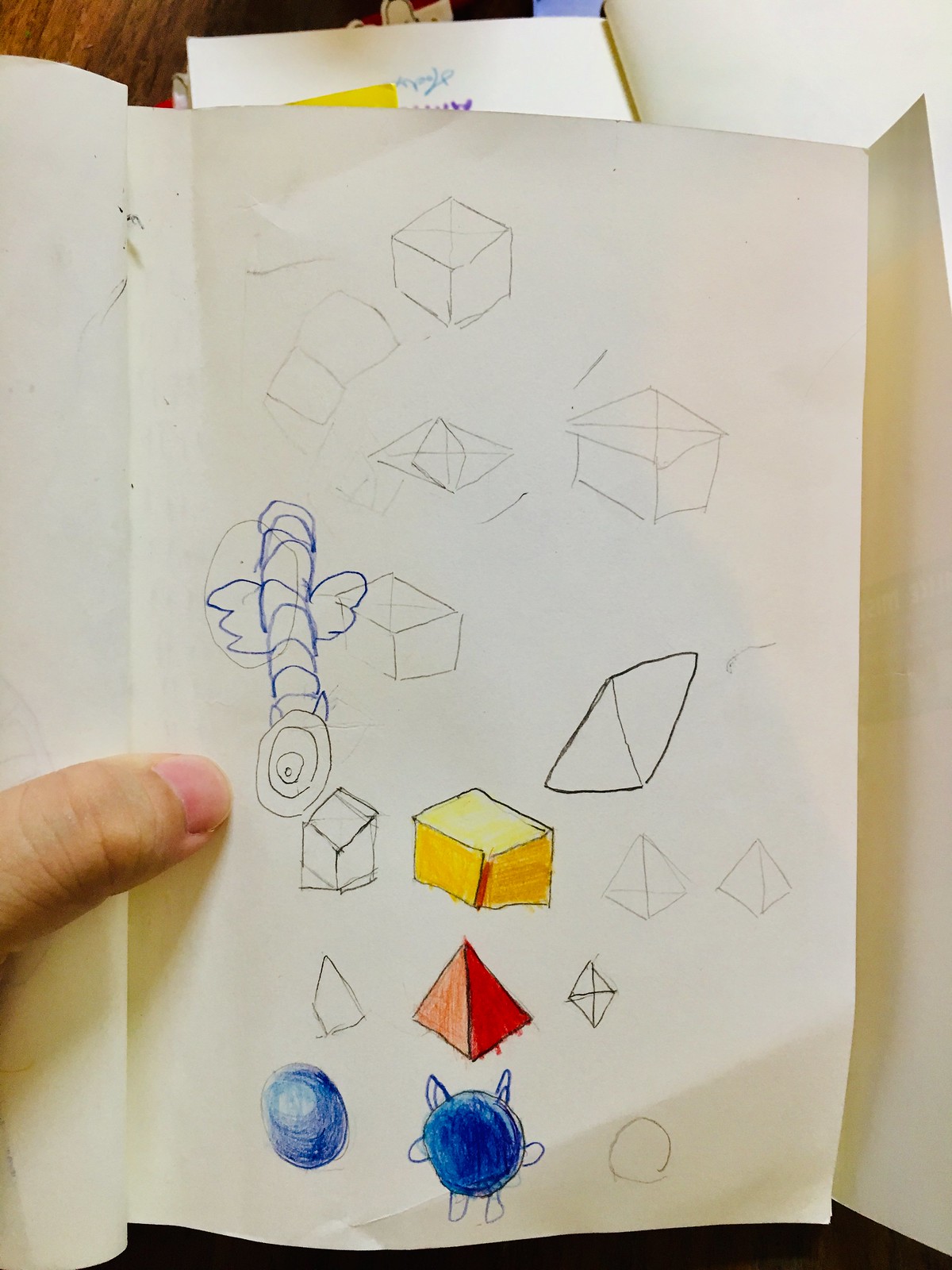A white piece of paper, held up by a fair-skinned male thumb, serves as the canvas for a collection of hand-drawn shapes and objects. Initially sketched in pencil, there is a three-dimensional square and another square with a smaller square on top, marked with an X. The medium transitions to pen or possibly marker, adding a mix of vibrant colors to the scene. One box is fully filled in with yellow, while another contains a red-colored triangle. A blue circle adorned with multiple notches stands out, alongside a solid blue ball, illustrating a playful and diverse range of artistic elements.